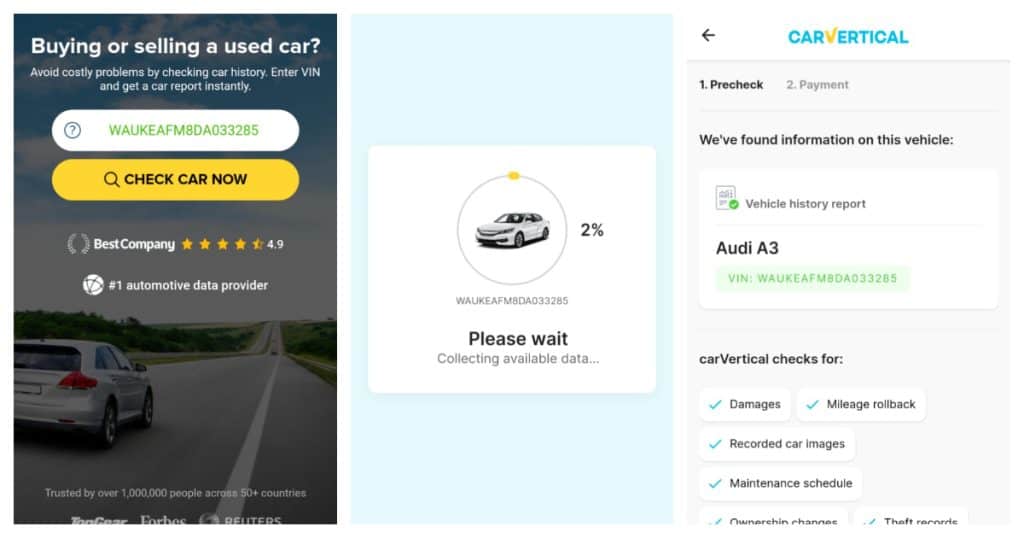The image depicts a detailed overview of a car history report service. On the left side, a blue vertical banner with a gold "B" and a black left-pointing arrow reads "CAR VERTICAL." Beneath it, the steps "1. Pre-checked" in blue and "2. Payment" in gray are listed. Below these steps, the text "We found information on this vehicle" is followed by "Vehicle History Report," accompanied by an icon resembling a square with dots and a green circle with a white check mark.

Black text indicates the vehicle is an "Audi A3" and a green shaded banner displays the VIN number. The section titled "Car Vertical Checks For" lists checks in white banners with black letters and blue check marks, including damages, mileage rollback, recorded car images, maintenance schedule, ownership changes, and theft records, though some are cut off.

In the middle of the image, a blue shaded area showcases a white car and the text "2%." Below the VIN-like code "WAUKEAFMA," the phrase "Please wait, collecting available data…" appears. On the left side, a shaded background picture of a highway features a four-door silver car driving, with fields on either side and an endless road ahead. Above this image, white text states "Buying or selling a used car? Avoid costly problems by checking car history."

Below, it instructs users to "Enter VIN and get a car report instantly," with a white input banner containing a green VIN number. A gold banner below the input area displays "Check Car Now" in black with a black search icon. At the bottom, the text "Best Company" in white is accompanied by gold stars with a rating of 4.9, and the statement "Number one automotive data provider" is prominently displayed.